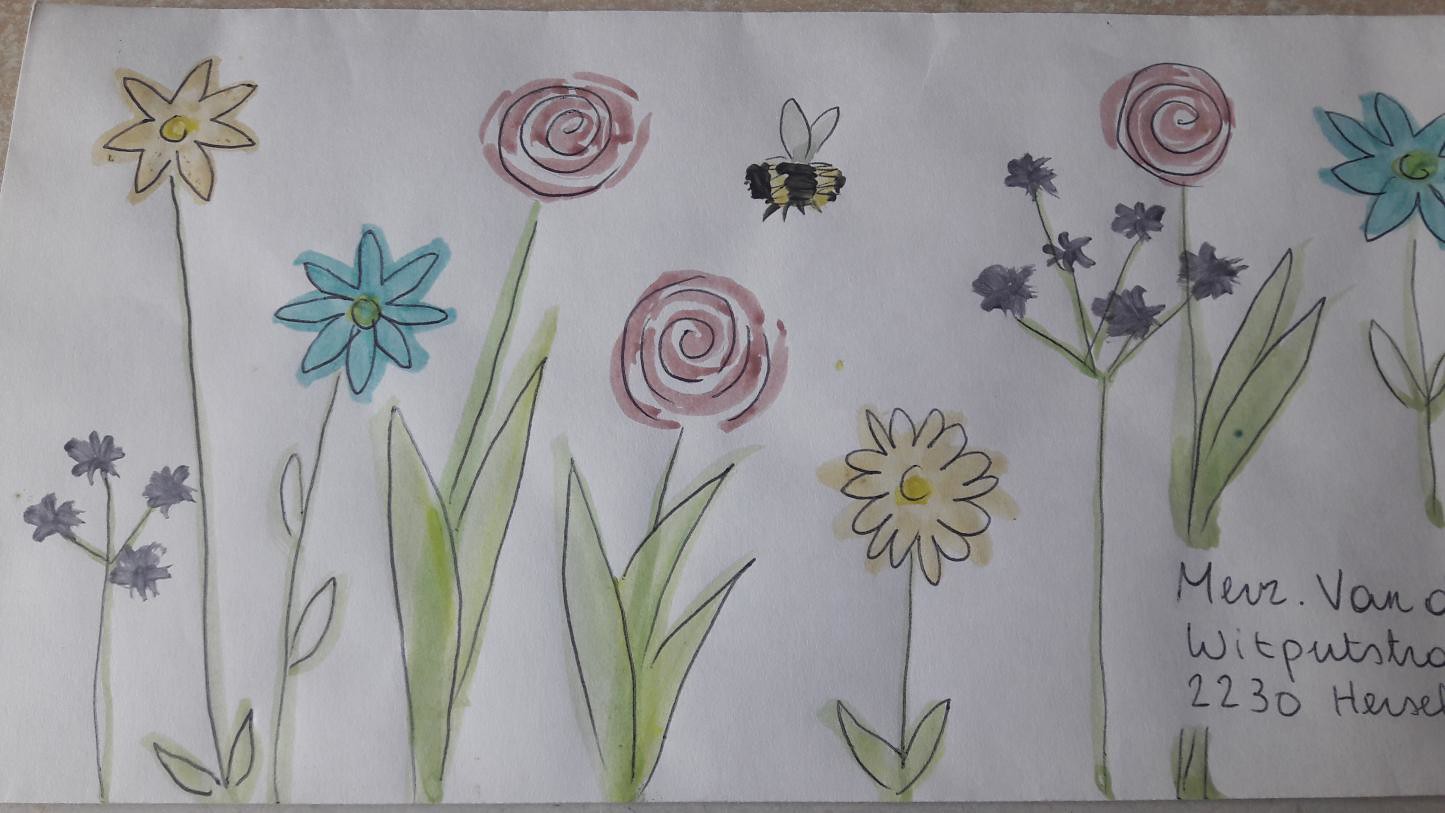This image depicts a hand-drawn, colorful arrangement of various flowers and a bee on what looks like a white envelope. Starting from the left, a small purple flower on a green stem splits into four blooms. Next to it is an orange-yellow star-shaped flower with two leaves at the bottom. A blue star-shaped flower stands to its right, slightly shorter. Following this is a taller red flower with petals resembling a cinnamon bun swirl and two long leaves, mirrored by a slightly shorter identical bloom next to it. A small yellow flower with two green leaves and a stem is next. Toward the right, another tall flower with six purple blooms on one green stem appears. Among these vibrant flowers, a black and yellow fuzzy bee with white wings is depicted flying to the left.

At the lower right corner of the envelope, an incomplete address is visible, reading: "M-E-V-Z. van V-A-N," followed by "W-I-T-P-U-T-S-T-R," and below that "2-2-3-0-H-E-R-S-E-L."